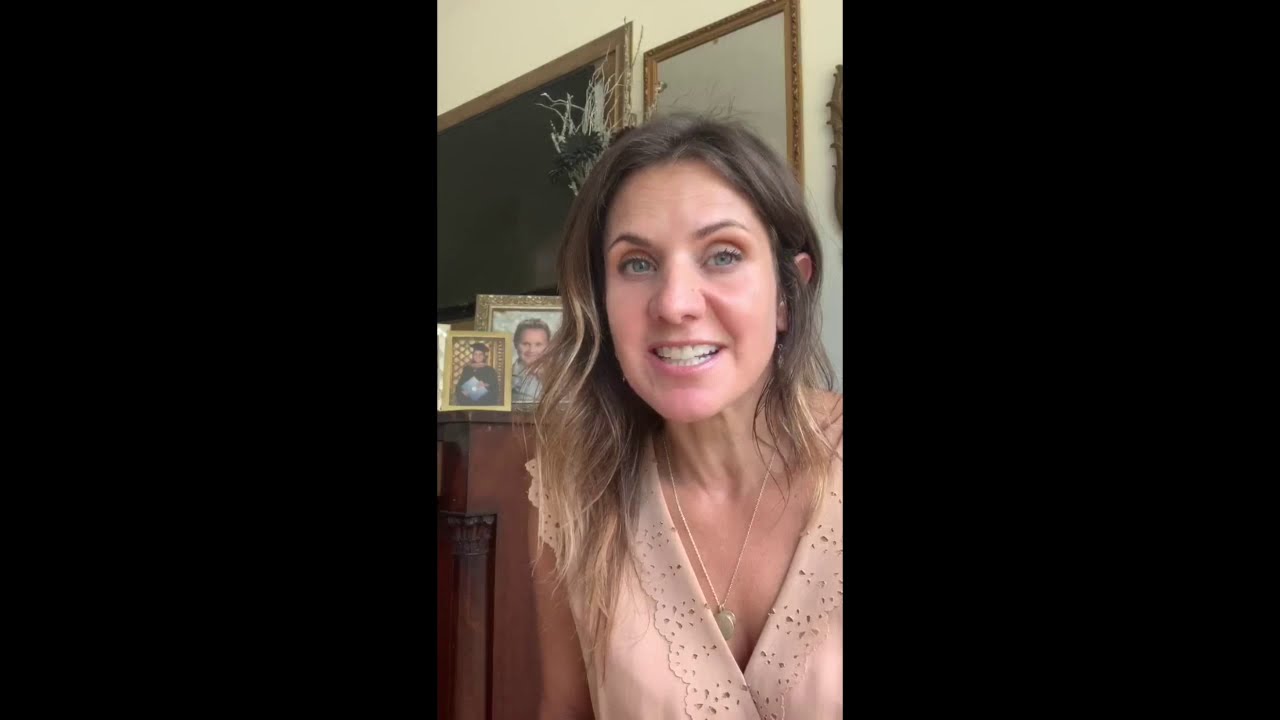The image shows a middle-aged Caucasian woman with sandy blonde hair that transitions to bleach blonde from her ears down to her bust line. She has softly arched brows and blue-green eyes. Her hair is parted in the center, with strands falling softly on either side of her face and over her shoulders, with her left ear partially visible as some hair is tucked behind it. She is seated in a living room and is smiling broadly, showing her teeth, and exudes a content demeanor. She is wearing a light tan, sleeveless v-neck blouse with lace trimming and a gold locket necklace. 

The room behind her features yellow-painted walls adorned with a large black chalkboard decorated with foliage, and a gold-rimmed mirror is directly behind her head. On the left side of the image, a wooden dresser holds two gold-framed photographs—one of a young Caucasian male child and another of a Caucasian female child in a black cap and gown, possibly a graduation photo. Another indiscernible object is observed to the right behind her head. The background of the image is mostly black, with the left and right thirds blacked out, drawing focus to the vibrant center where the woman is positioned.

Overall, this detailed depiction combines shared elements from different descriptions to provide a vivid representation that emphasizes the woman's appearance and the living room's distinctive features.